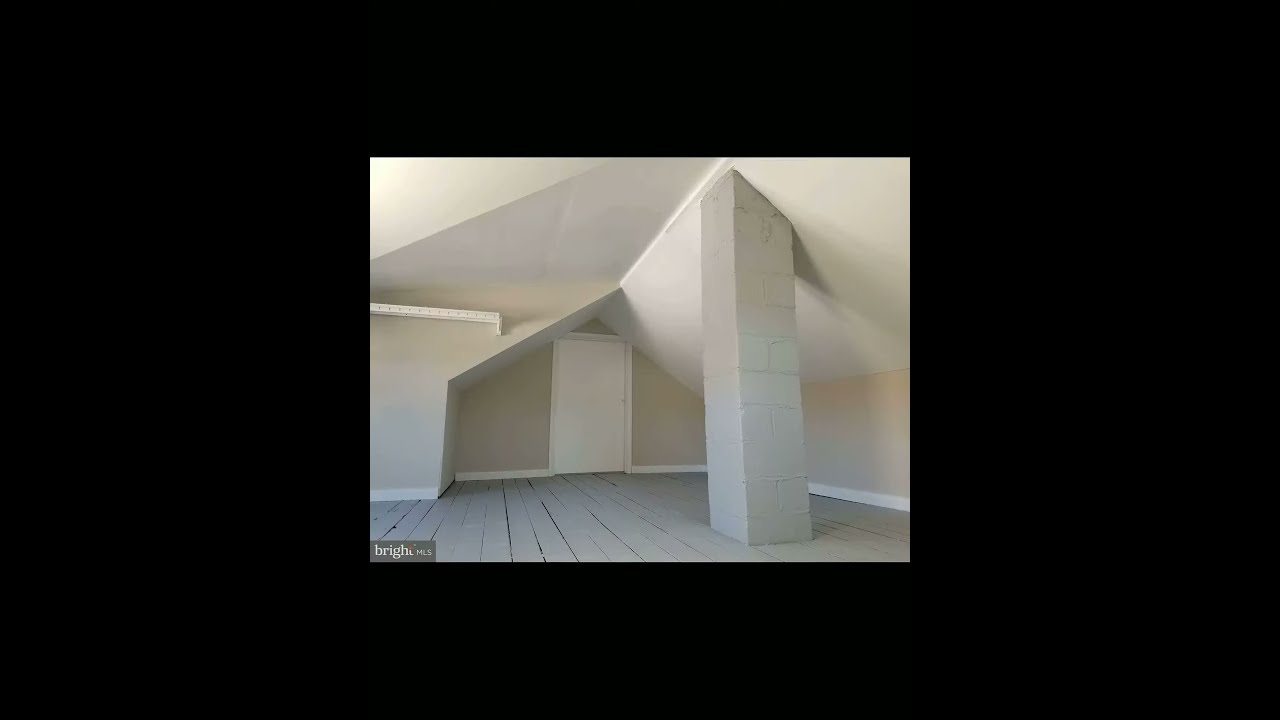The image depicts an uncluttered and vacant attic room, distinguished by its vaulted ceiling that reveals the pitched roof lines. The floor consists of gray painted wooden planks, while the walls are painted a light beige with white trimming, including the baseboards and the ceiling edges. A closed, seemingly short white door is visible in the background, adding to the room's minimalist aesthetic. On the right side, a white-painted structure, likely a chimney made of hollow tile brick, extends from floor to ceiling. The room is devoid of any furniture, decorations, or personal items, giving it a modern, pristine, and starkly white appearance. In the lower left corner, against a thick black background, there is a logo or inscription in white lettering that reads "Bright MLS," suggesting it is associated with a real estate firm.